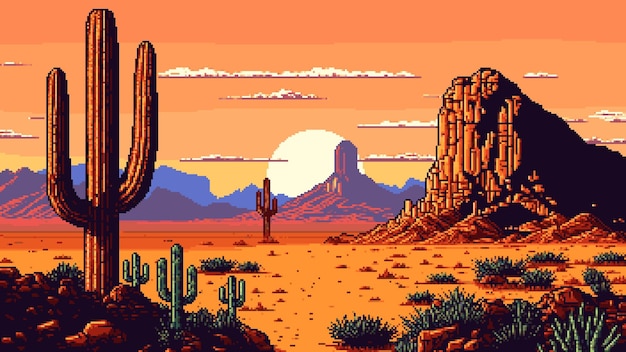A vibrant cartoon depiction of a Western landscape, featuring a striking orange sky that gradients into a lighter orange hue, crowned by a large, glowing white sun. Long, thin white clouds stretch across the horizon, highlighting the scene's surreal beauty. In the background, purple mountains intermingle with blue tones, providing a majestic contrast to the foreground. The land is a rich palette of dark and lighter brown sands, interspersed with patches of green vegetation. A massive brown rock formation dominates the landscape, surrounded by smaller rocks and sandy terrain. Scattered across the scene are small green cacti, with one prominent brown cactus showcasing two large arms, further accentuating the rugged charm of this Western vista.